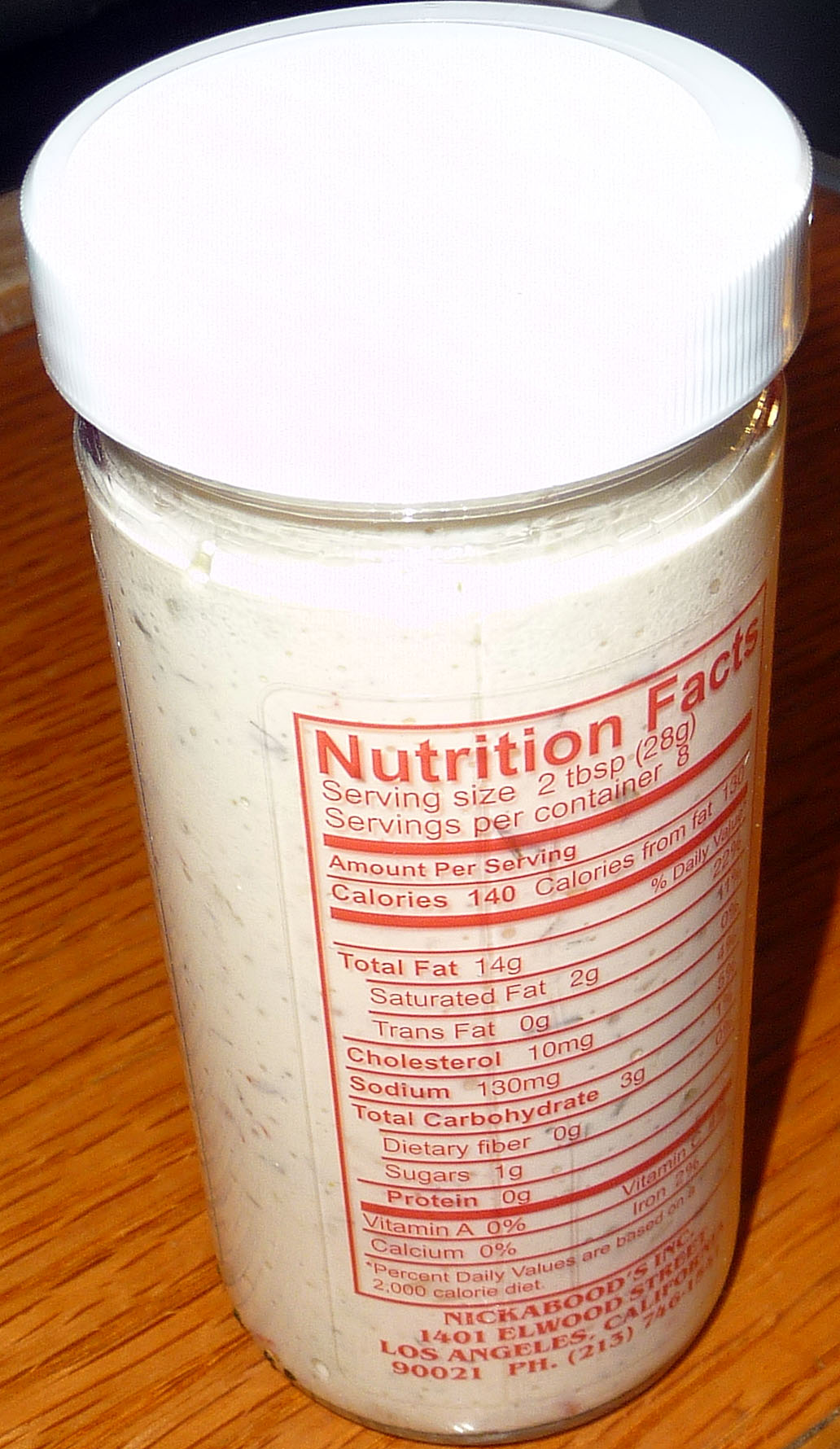Close-up of a transparent container, possibly made of glass or plastic, showcasing its back side. The container features a white twist-off cap and appears to hold a condiment such as horseradish, hollandaise sauce, or mayonnaise. Visible on the back are detailed nutrition facts, including a serving size of two tablespoons, 140 calories per serving, and 14 grams of total fat. The bottom of the label indicates the manufacturer as Nickel Boobs Inc., located at 14 Egglewood, Elwood, California.